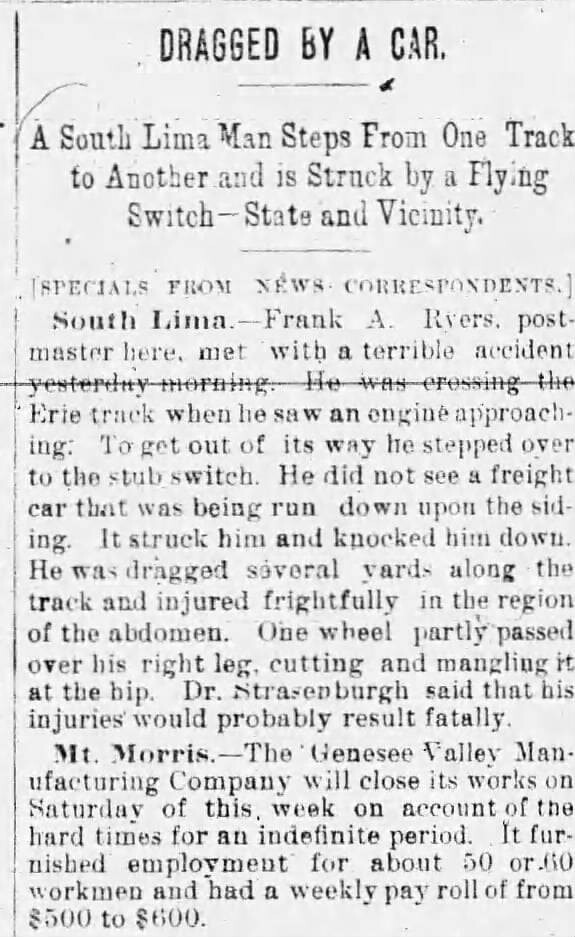This image appears to be an old, worn scan of a Xeroxed newspaper clipping, marked by flaws such as horizontal lines and scratches in the text. The headline, in capital letters, reads "DRAGGED BY A CAR," with a thin line underneath. Below this, the sub-heading states, "A South Lima man steps from one track to another and is struck by a flying switch - state and vicinity." A bracketed note follows, saying "SPECIALS FROM NEWS CORRESPONDENTS." The main story, in bold, begins with "South Lima," likely referring to South Lima, Ohio. It chronicles a tragic incident involving Frank A. Reiers, the local postmaster, who was struck and dragged several yards by a freight car after stepping onto a stub switch to avoid an oncoming engine. The detailed account mentions severe injuries to his abdomen and right leg, with dire predictions from Dr. Strassenberg regarding his survival. In the subsequent bolded paragraph, the article diverges to report economic hardships faced by the Genesee Valley Manufacturing Company in Mount Morris, which plans to close indefinitely, impacting about 50-60 workers and a weekly payroll of $500-$600. The juxtaposition of these disparate topics highlights the fragmentary nature of the clipping.